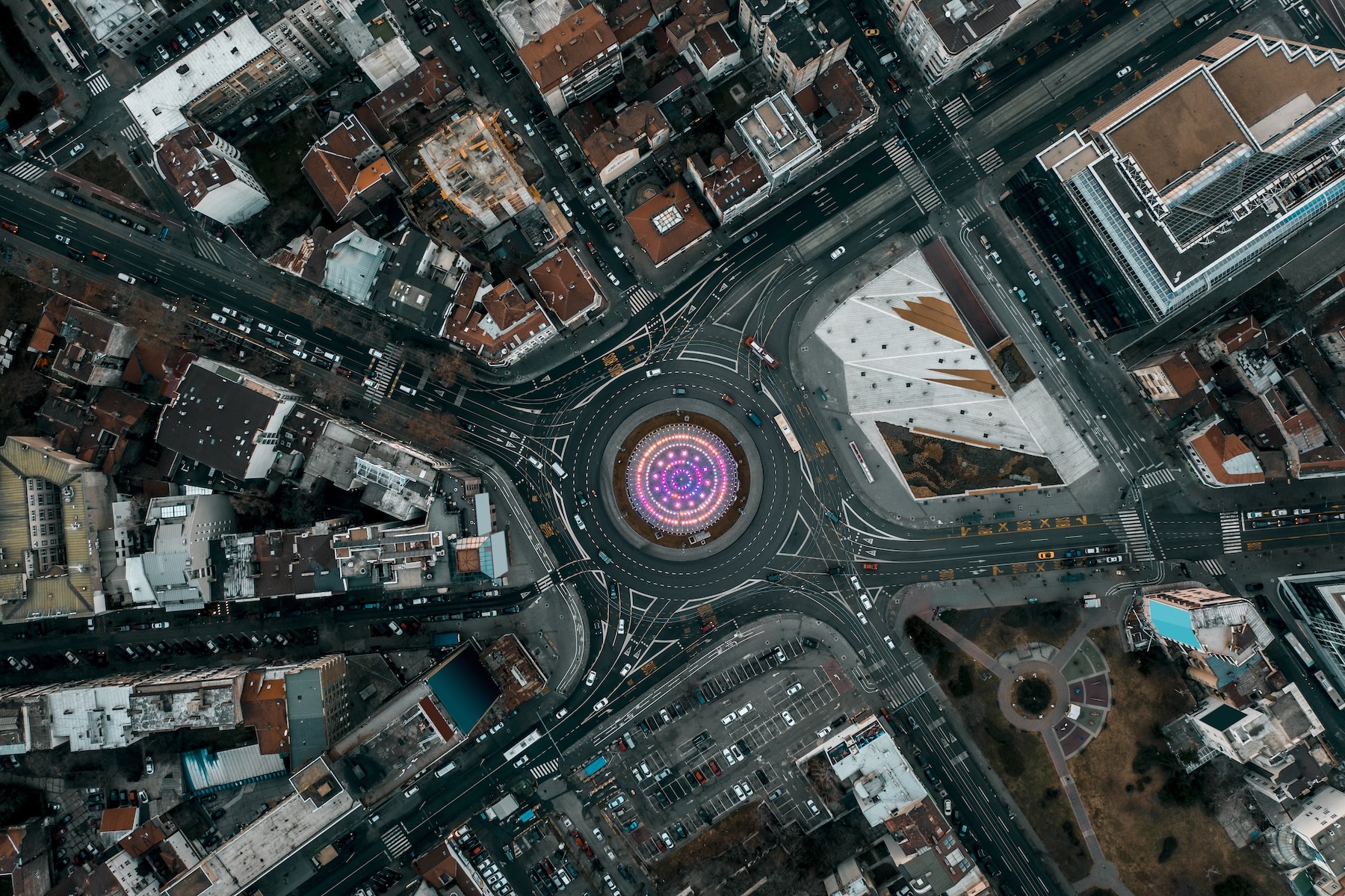This aerial photograph, taken from high above, depicts a bustling cityscape centered around a striking, circular area that appears to be a major intersection or roundabout. The roundabout is multi-layered with distinct, vibrant colors: an outer dark blue ring, followed by a glowing neon orange ring, and a series of smaller circles in pink and bright white, some of which are glowing dots. Within the central circular feature, there's a series of rings showcasing a palette of green, purple, pink, blue, and orange, gradually leading to a prominently glowing green center.

Surrounding this colorful focal point is a mix of urban elements: streets teeming with a variety of vehicles, including cars and trucks in whites, grays, and blacks, along with parking lots. The layout reveals a clear grid pattern characteristic of a city, comprising both commercial buildings with flat white roofs and residential areas. To the central right of the image, a large building with a flat white roof stands out amongst blocks of smaller structures, possibly hinting at a combination of commercial and residential uses. Notably, the city features patches of green grassy areas, possibly parks, though some grass appears brown, indicating a winter season. The image captures a dynamic and detailed snapshot of the city’s infrastructure and urban life.